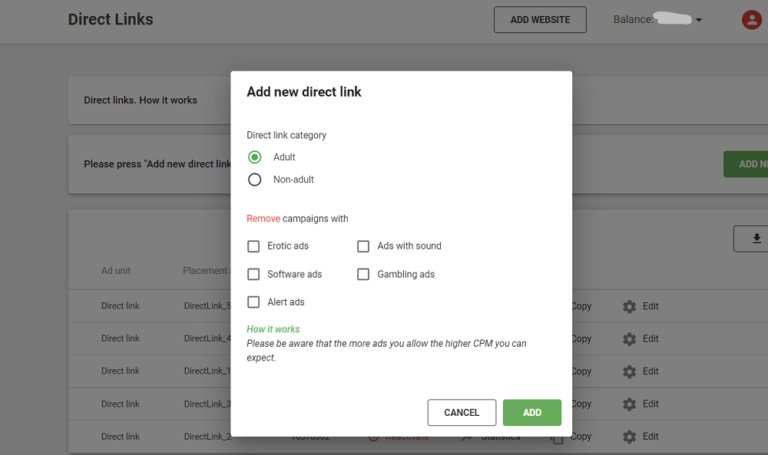**Caption for Image:**

In the image, the main webpage is grayed out due to an overlaying pop-up window. The grayed-out page includes options titled "Direct Links," "How It Works," "Pre," "Plus," "Add New Direct Link," with some sections obscured or edited out, particularly the "Balance" section. 

Centrally, a prominent white pop-up box is displayed, which dominates the screen. At the top of this box, the text "Add New Direct Link" is presented in bold black letters. Below, in smaller, regular black font, the pop-up offers a choice for "Direct Link Category" with two options: "Adult" and "Non-Adult." The "Adult" option is selected, indicated by a green-highlighted circle.

Further down, red text marked "Remove" is shown, and beside it, black text reading "Campaign with." Each accompanying checkbox offers categories such as "Erotic Ads," "Software Ads," "Alert Ads," "Ads with Sound," and "Gambling Ads." All of these checkboxes are accompanied by descriptive labels. At the bottom of this list, in green text, there is a "How It Works" section.

Finally, the pop-up includes two action buttons at the bottom: "Cancel" and "Add."